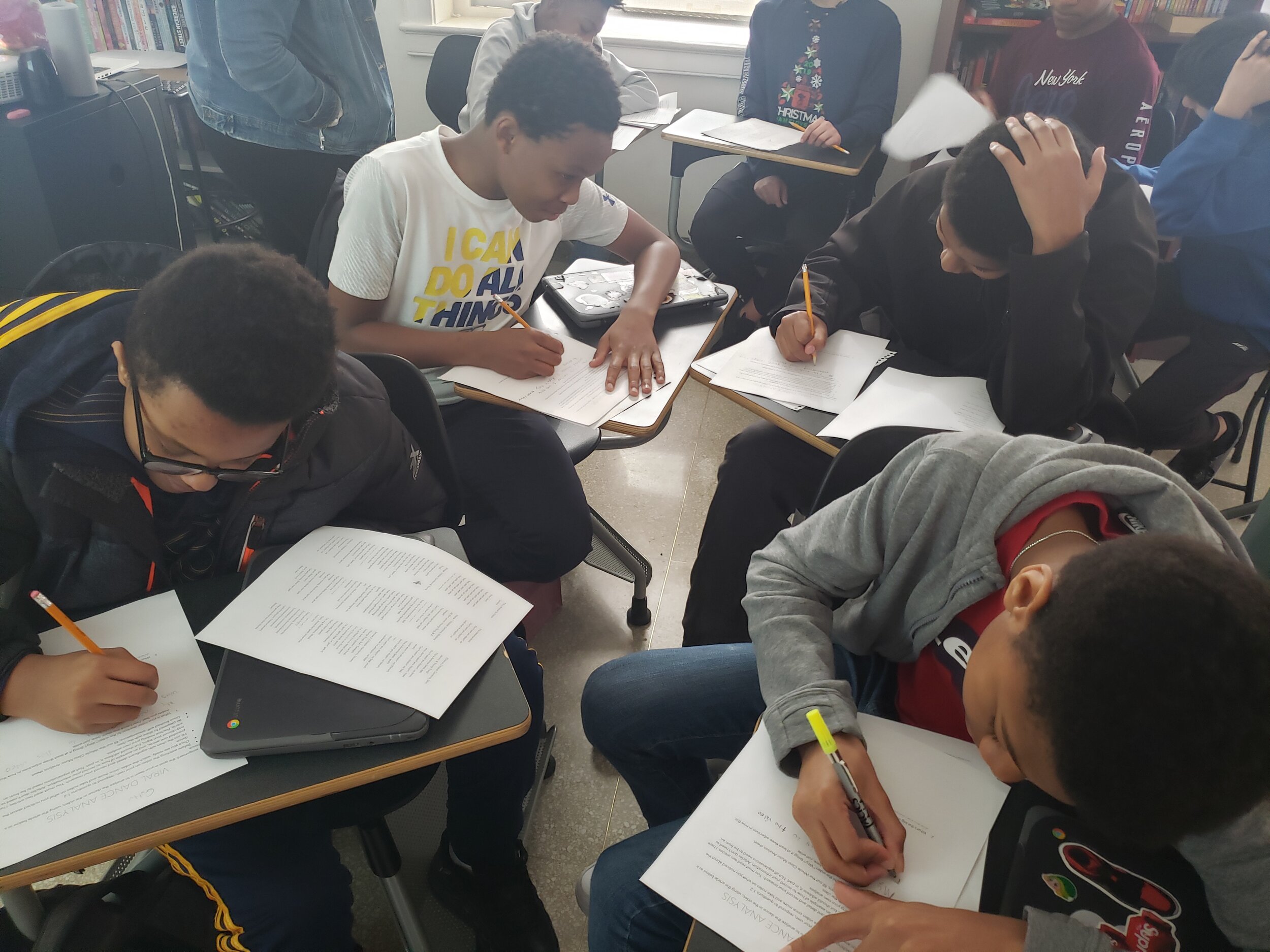In this top-down image, around ten students are dispersed throughout a classroom, each sitting at mismatched desks that lack any structured arrangement. Most desks hold multiple pieces of paper and binders, with a few students also utilizing laptops, likely Chromebooks. The students, predominantly of varying black skin tones, are deeply engrossed in their work. At the center of the scene is a boy in a white shirt with yellow and black letters stating "I can do all things," who is glancing at the paper of the student in front of him. Towards the bottom right, another student in a gray sweatshirt and red shirt unique for using both a yellow marker and a number two pencil is also busy writing. The background reveals some students in conversation, possibly with a standing teacher, while natural light casts a hazy glow over the room, further softening the scene.